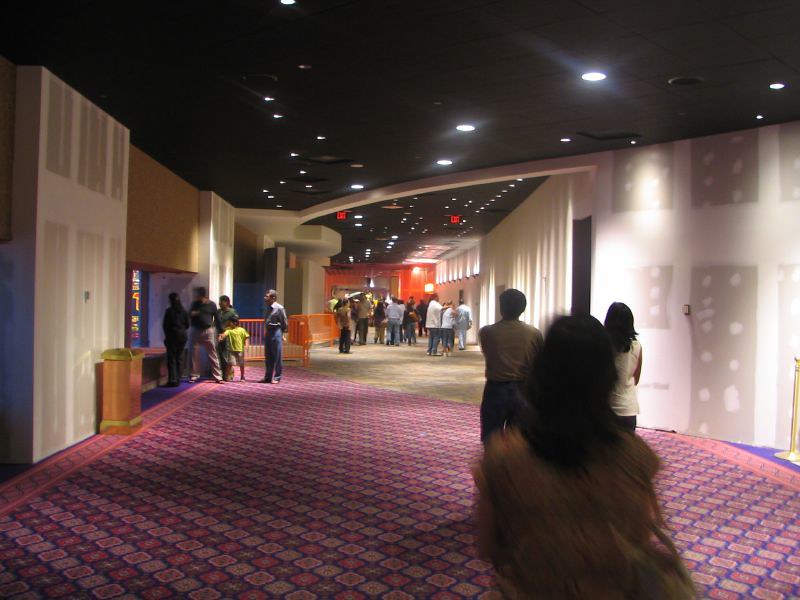This image depicts an indoor walkway, likely within a convention hall or museum-like space, filled with a casually dressed crowd leisurely exploring their surroundings. Prominent in the foreground is a woman with long dark hair, wearing a yellowish-gold blouse, standing on a vibrant carpet of purplish, red, and pinkish hues. As the carpet transitions to a light greenish color, the eye is drawn to a variety of details: a message board on the left side with several people studying what appears to be a map, a large doorway with white doors accompanied by a small pedestal near it, and structural elements such as a diagonal beam overhead. The area is brightly lit with overhead lights, and the walls are mostly bare, suggesting the displays and structures within the hall were added for a temporary event. In the background, an orange railing can be seen behind some of the visitors, and the floor gives way from carpeting to concrete, enhancing the bustling ambiance of the convention-like environment.